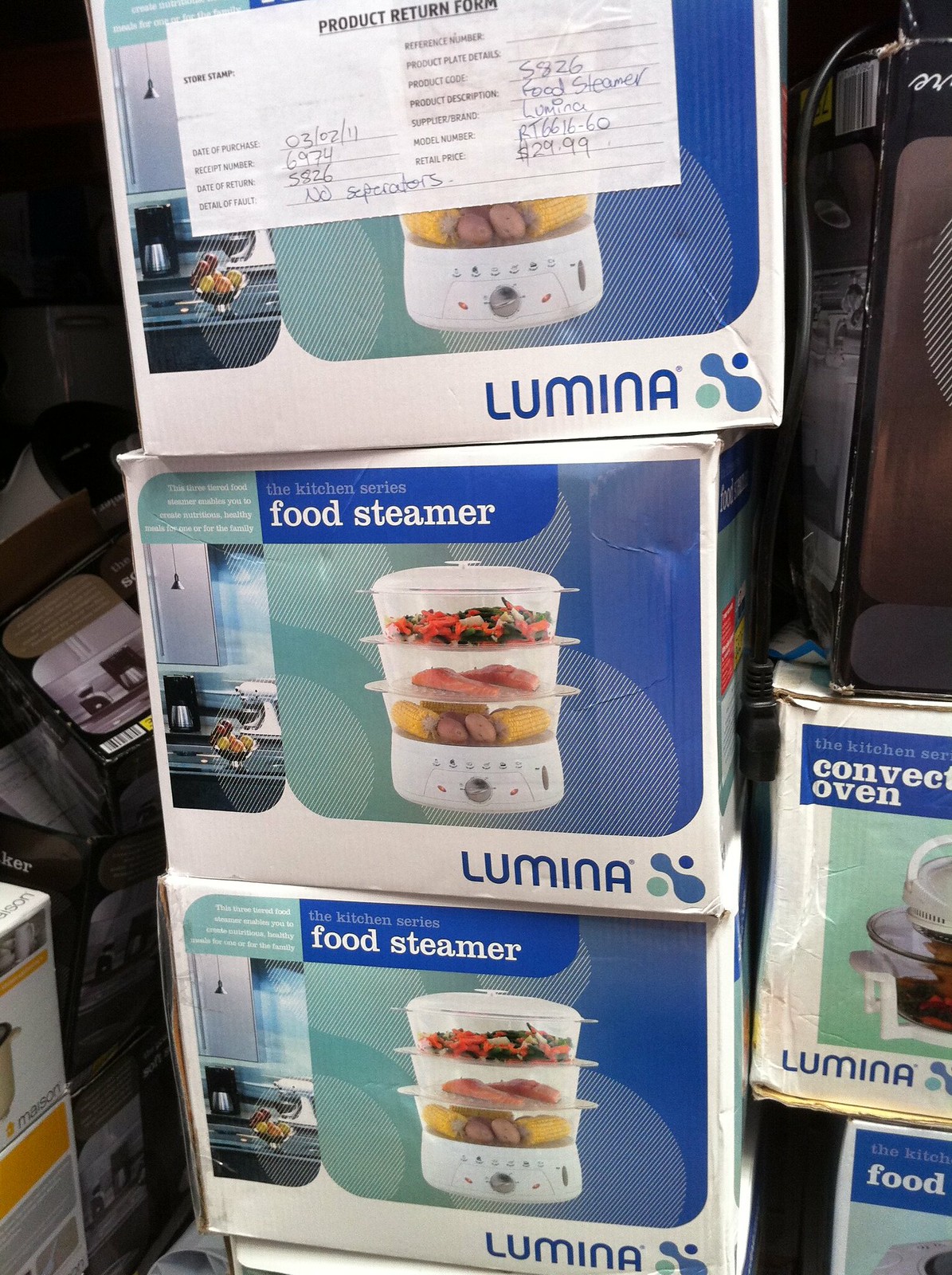The image depicts a cluttered storage area filled with numerous items, prominently featuring multiple boxes of Lumina-branded food steamers. In the center, there are three boxes of the Lumina food steamer stacked vertically, displaying a white cylindrical device with three transparent layers, each containing food items such as vegetables and meat. The boxes are primarily blue and white. On the right side, there are two additional boxes; one of them labeled as a convection oven, partially hidden under other miscellaneous items. One topmost box has stickers indicating it is a product return form, noting details such as a return date of March 2, 2011, appliance model number RT6616-60, and a retail price of $29.99. The surrounding area is chaotic, with various other boxes and items cluttering the space, adding to the overall sense of disorder.